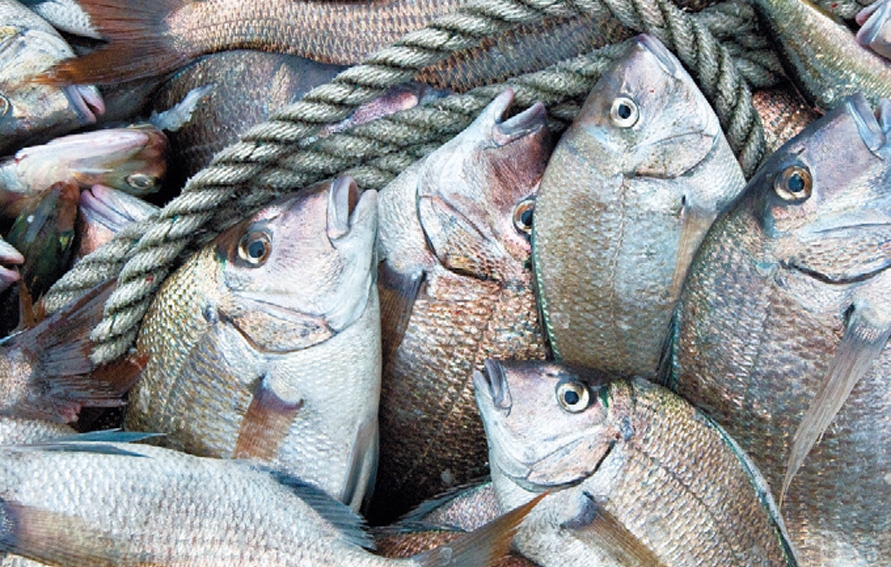This close-up photograph captures a dense pile of fish, their silvery scales shimmering with hints of rainbow-like iridescence, interspersed with shades of green and brown. The dead fish lie on a rough burlap surface, their large eyes wide open and mouths slightly ajar, indicating they were recently caught. A thick, twisted rope zigzags through the composition, seeming loosely interwoven among the fish but not tied around any specific one. In the center, a nearly whole fish is prominently visible, surrounded by others stacked and overlapping in various directions. Notable details include a large fish tail in gold-brown color at the top left corner, and another fish body covered partially by the rope toward the right. The overall scene is chaotic, with no uniform pattern to the arrangement of the fish, adding to the raw, natural feel of the image.